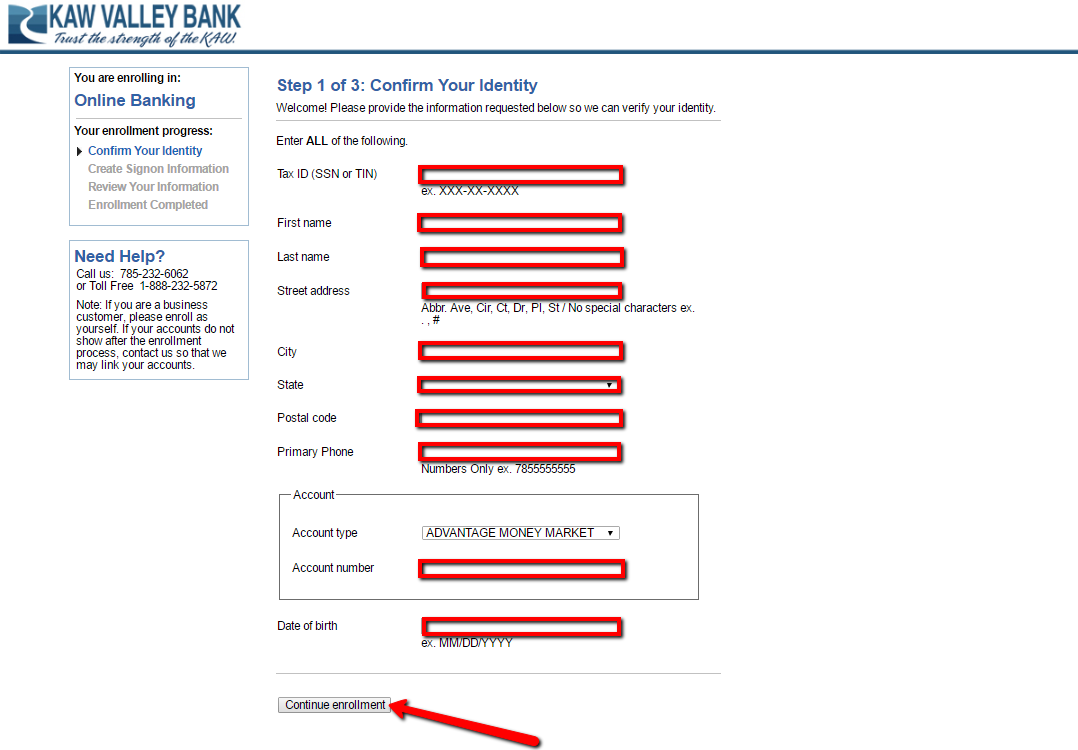This image captures a webpage from Kaw Valley Bank, prominently showcasing the bank's name in capital letters written in dark blue ink at the top left corner. Alongside the name is the tagline, "Trust the Strength of the Kaw." Next to the title is a blue logo featuring a white river flowing through it.

The webpage is an enrollment form for online banking, specifically showing Step 1 of 3, focused on confirming the user's identity. The form extends a welcoming message and asks the user to provide various pieces of information to verify their identity. 

The instructions emphasize that all fields must be filled out, with the word "ALL" capitalized for emphasis. The requested information includes:

- Tax ID number
- First name
- Last name
- Street address
- City, state, and postal code
- Primary phone number

Each field is accompanied by a white rectangle outlined in red, which users can click on to type their information. Below that, the form asks for account details, with "Account Type" pre-selected to "Advantage Money Market." Another red outlined box awaits the account number, followed by a field for the date of birth.

A large red arrow points towards a button at the bottom of the page labeled "Continue Enrollment," which guides the user to proceed to the next step of the enrollment process.